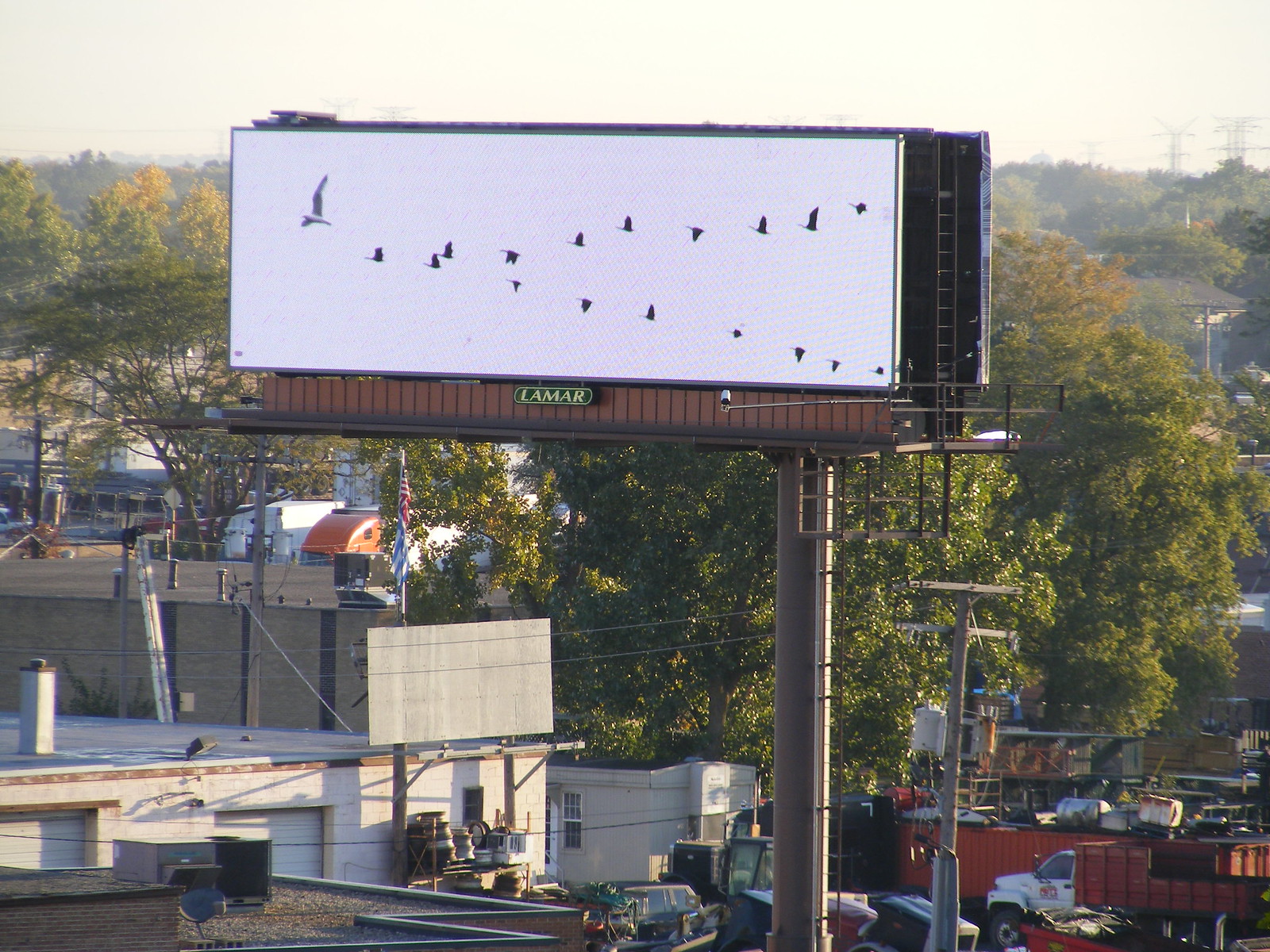In this urban industrial setting, a prominent billboard towers over the scene, mounted on a substantial stone pole. The billboard features a striking image of a flock of birds against a stark white background. Positioned on the top left is a leading white bird, followed by black birds in a V formation. Below this flock, the word "Lamar" is prominently displayed. Surrounding the billboard are power lines, various trees, and the tops of buildings. The streets below are dotted with semi-trucks and dump trucks, characterized by white cabs and red cargo areas. The sky in the background, tinged with a hint of yellow, suggests the approach of dusk. This mix of industrial elements and urban environment captures a moment teeming with everyday life and activity.